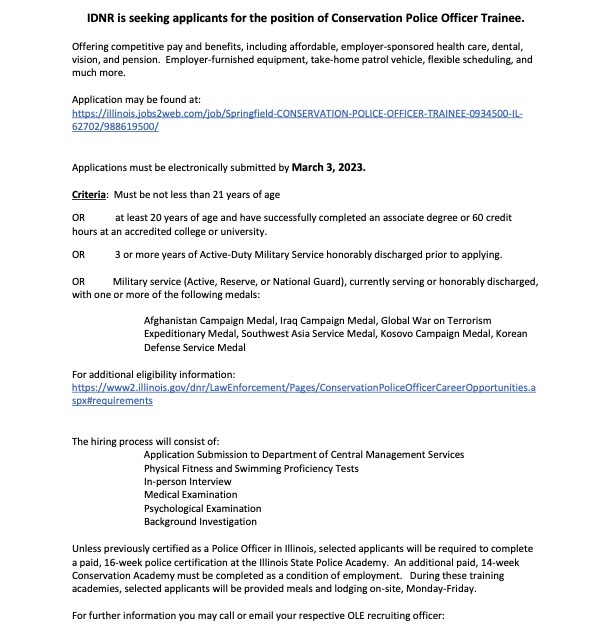The image depicts a webpage with detailed information about a job opening for a Conservation Police Officer Trainee at the Illinois Department of Natural Resources (IDNR). At the top of the page, a bolded black text heading reads, "IDNR is seeking applicants for the position of Conservation Police Officer Trainee." Immediately below, on the left-hand side, a list of benefits is outlined, including competitive pay and benefits, affordable employer-sponsored health care, dental, vision, a pension plan, employer-furnished equipment, a take-home patrol vehicle, flexible scheduling, and more. 

Further down the page, it indicates in blue text that applications can be found online at a provided website. Slightly above the center of the page, the text specifies that electronic submissions of applications must be made by March 3rd, 2023, with the date prominently bolded. Below this, requirements for applicants are detailed, stating candidates must be at least 21 years old, or 20 years old if they have successfully completed an associate degree or 60 credit hours from an accredited college or university. Alternatively, applicants can qualify with three or more years of honorably discharged active duty military service or current service/honorably discharged status in the active reserve or National Guard.